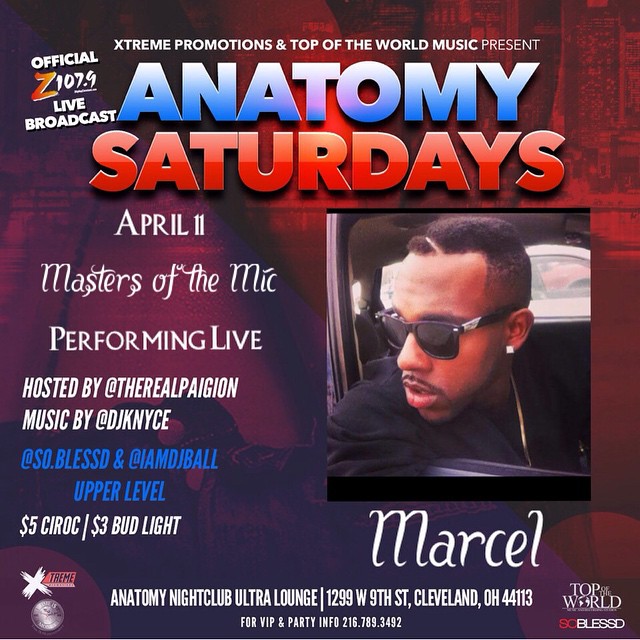This square-shaped advertisement poster for Club Anatomy features a shadowy background with a red and purple overlay, making the image somewhat indistinct. Overlaying the background in white text at the top, it reads "Extreme Promotions and Top of the World Music Present." Below this, prominently displayed, are the words "Anatomy Saturdays" with "Anatomy" in blue and "Saturdays" in red. 

To the left, the poster advertises an "Official 107.9 Live Broadcast". Beneath "Anatomy Saturdays," also in white text, it announces "April 11th Masters of the Mic performing live," hosted by "@TheRealPagan" with music by "@DJNice." Further down in blue, it mentions DJs "@SoBlessed" and "IAMDJBall" for the upper level. A beer special note follows, detailing "$5 Ciroc" and "$3 Bud Light" offers.

On the right side of the poster, there is a photo of a gentleman wearing sunglasses, a black sweatshirt, and a gold chain necklace, looking out from a vehicle window. Beneath his image, "Marcel" is printed in white text. Across the bottom of the ad, "Anatomy Nightclub Ultra Lounge" is written in white, along with the address on West 9th Street, Cleveland, Ohio 44113, and contact info for VIP and party details at 216-789-3492. The corners feature logos for "Extreme Promotions" and "Top of the World Music," though they are partially obscured.